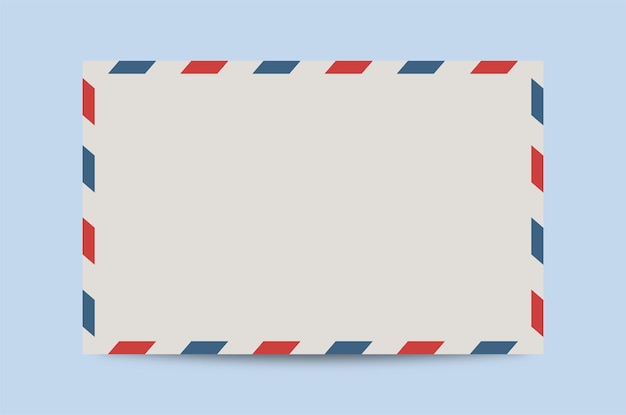This image features a white rectangular envelope-like shape set against a light sky-blue background. Surrounding the perimeter of the rectangle is a distinctive border composed of alternating red and blue trapezoidal segments, separated by white spaces, creating a repetitive pattern that runs along all four edges. The interior of the rectangle remains entirely blank, emphasizing its simplicity. Additionally, a slight black shadow is visible at the bottom center, enhancing the three-dimensional effect of the image.